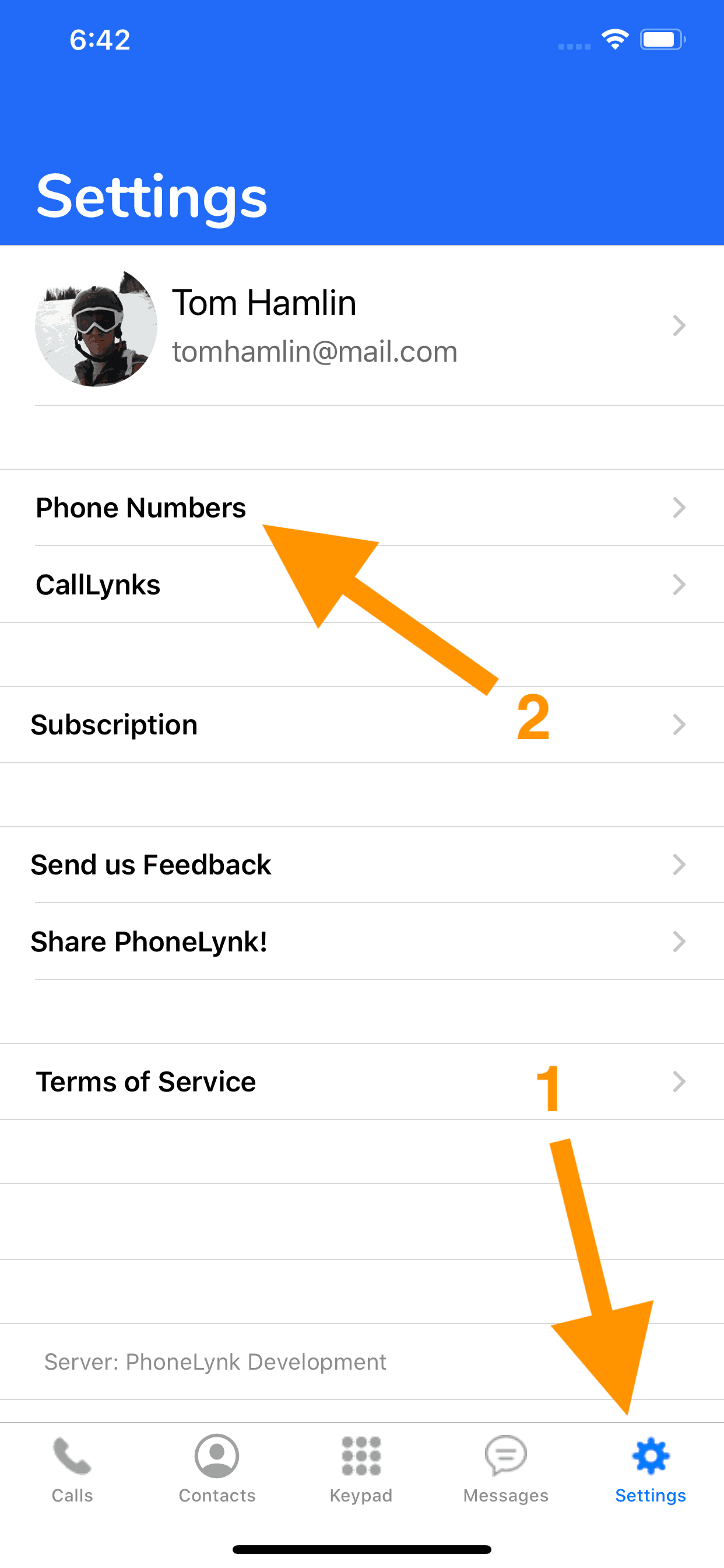The image depicts a settings section on a mobile application, which appears to be either a contacts app, a phone management section, or a texting app. At the top of the screen, the name "Tom Hamlin" is clearly displayed, followed by the email address "tomhamlin@mail.com". Directly below this, there's a profile picture showing an individual dressed in snowboarding gear.

The section lists various options including:
- Phone Numbers
- Call Links
- Subscription
- Send Us Feedback
- Share Phone Link
- Terms of Service

Two prominent gold arrows are used as highlights within the image. The first arrow, labeled with the number "2", points towards the "Phone Numbers" option. The second arrow, marked with the number "1", is located at the bottom right corner, directing attention to the settings icon. These arrows are quite large and set to draw attention to these specific elements within the interface.